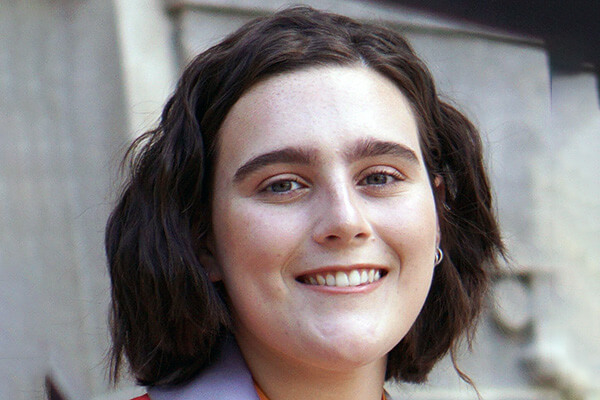The photograph features a young white woman with thick, wavy dark brown hair that reaches just above her shoulders. She has thick eyebrows and brown eyes, and is smiling warmly, displaying her upper teeth. Her lips are slightly colored, hinting at light makeup. She wears a couple of silver hoop earrings. Her outfit includes a blue or light purple overshirt with a red shirt underneath, and the picture captures her face and neck, stopping where her neck ends. The background shows a blurred, gray cement structure which suggests she is outdoors, with one side of her face illuminated by sunlight as she looks directly into the camera.